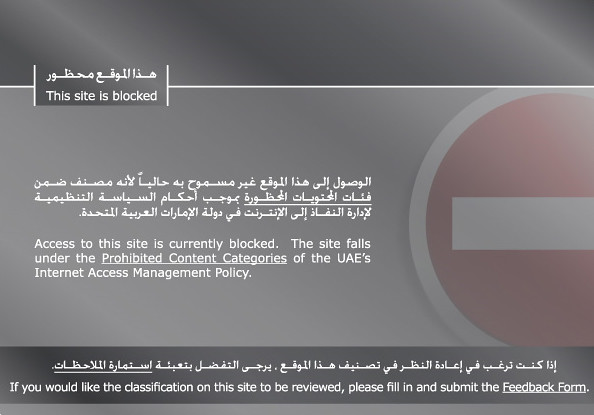The image depicts a screenshot of a webpage displaying an error message in both Arabic and English. The background is grey, with a dark top section and a lighter grey bottom section. At the top left in Arabic, it states that the site is blocked, followed by an English translation underneath saying, "This site is blocked." Further down, more Arabic text appears with the English translation beneath it, "Access to this site is currently blocked. The site falls under the prohibited content categories of the UAE's Internet Access Management Policy." To the right of this text is a faded red circle with a white border and a horizontal white bar across the center, indicating prohibition. The bottom section of the page has additional Arabic text with English text underneath it, stating, "If you would like the classification on this site to be reviewed, please fill in and submit the feedback form." Overall, the image clearly indicates that the webpage access is restricted based on the UAE's Internet regulations, and provides instructions for requesting a review of the site's classification.